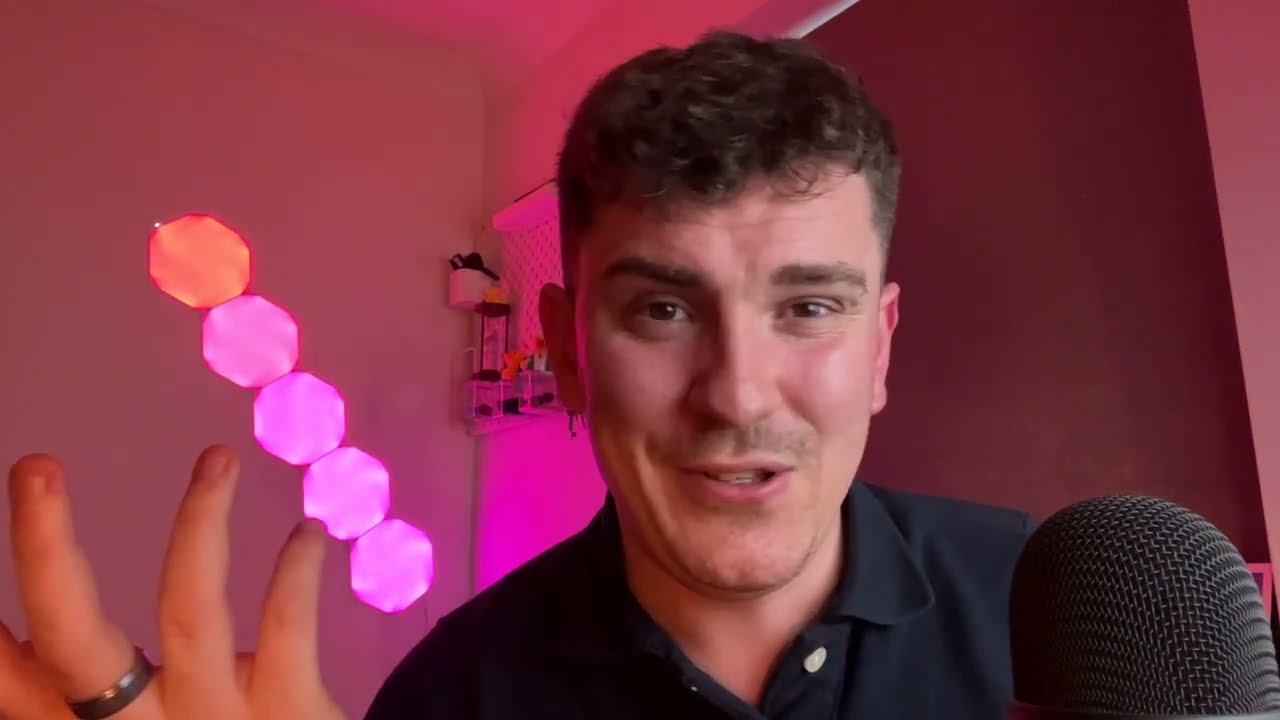The image is a close-up photo of a man, prominently positioned just right of center, showing his head, shoulders, and part of his upper torso cut off just below the chest. He has short, curly, brown hair, and is in the early stages of growing a thin mustache. His mouth is slightly open, suggesting he is in the middle of speaking, and he gazes directly ahead. The man is dressed in a dark-colored, collared shirt, presumably a polo or blue shirt.

In the image's bottom right corner, there's a large black microphone positioned in front of him, indicating he might be recording a podcast or speaking into the microphone. His right hand is raised and visible at the bottom left of the photo, showing three fingers and a ring on the left-most finger. Above his hand, a series of hexagonal shapes ascend diagonally towards the left; the four at the bottom are pink, while the top one is orange.

The background comprises various shades of pink and red. To the left of the man, the wall is mauve, transitioning to a pink area directly behind him, visible over his left shoulder, which contains some hangings. More to the right, the backdrop shifts to a crimson-colored wall. Additionally, behind his right shoulder, there's a rack-like structure holding small objects. Pink lighting elements add a soft, ambient glow to the image, emphasizing the monochromatic and colorful theme of the room.